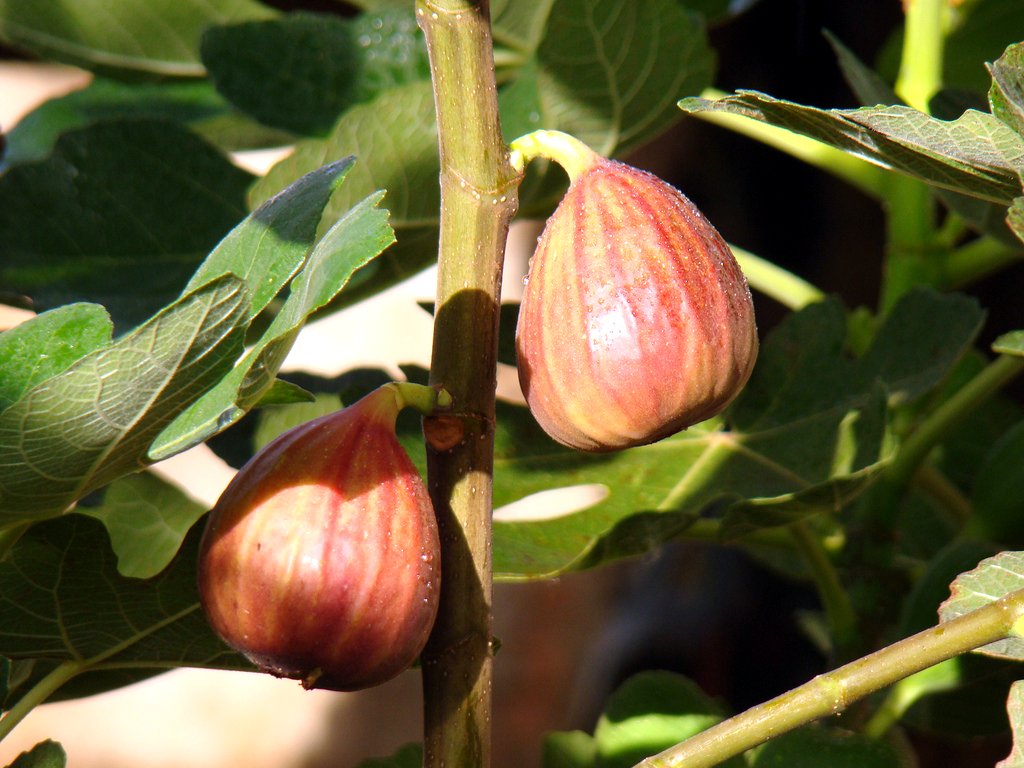This close-up photograph captures a detailed view of a plant's light brownish-green stalk, prominently displaying two hanging pods or fruiting bodies, one on each side. The pods, distinguished by their reddish-pinkish hues that merge into orangish-yellowish shades, appear rounded and somewhat oval-shaped towards the top, transitioning to a more circular shape at the bottom. The intricate texture and color of these pods suggest they are in an early stage of development, making it challenging to identify whether they are fruits, vegetables, or flowers. The dense green leaves form the background, with their pointed tips softly illuminated by natural light. Additionally, a smaller branch extends to the right off the main thick stem, contributing to the complex structure of the plant. The entire scene is set against a white surface, emphasizing the vibrant color contrast and fine details of the plant's components.